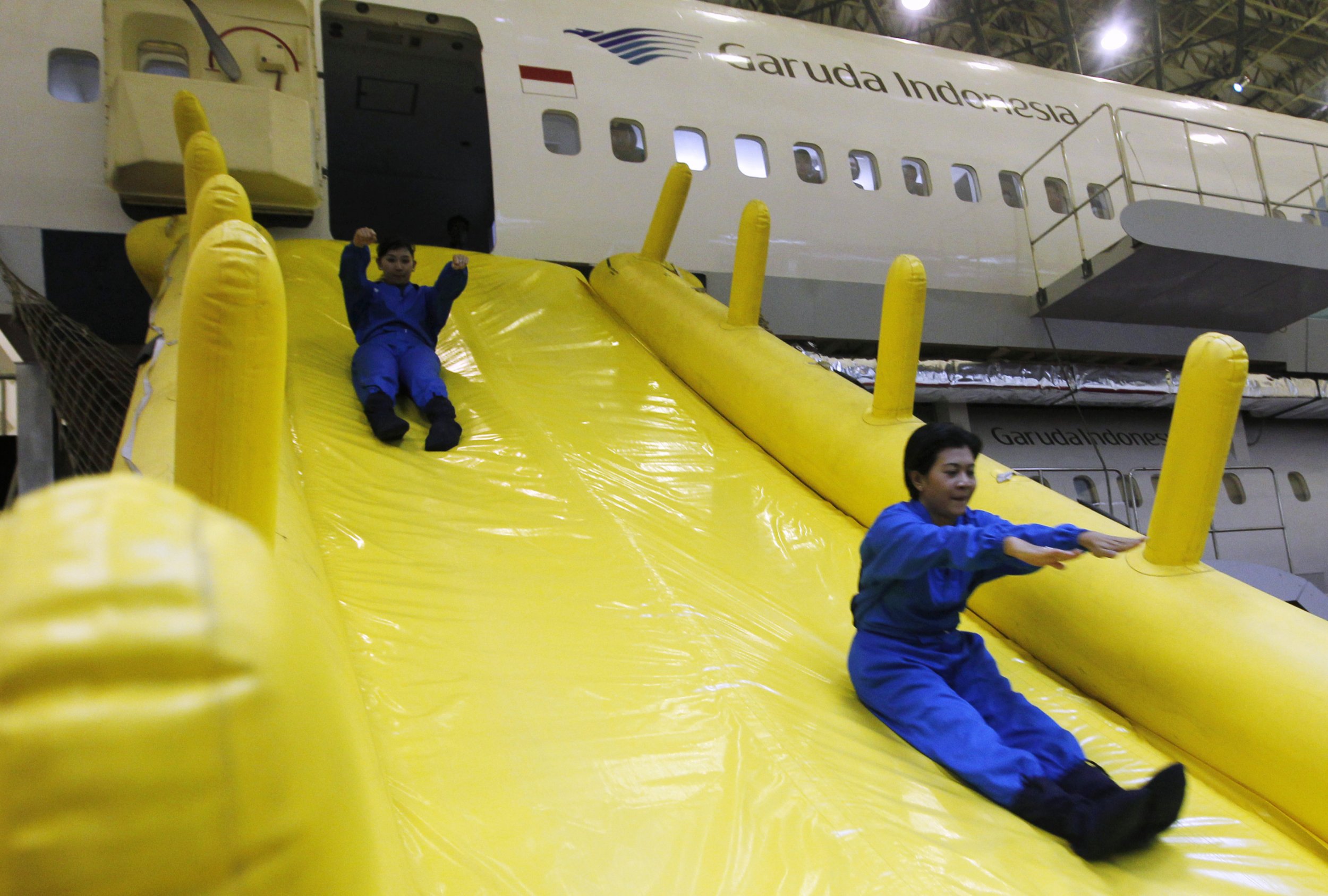The photograph depicts a detailed scene inside a large warehouse or hangar, showcasing a white airplane with "Garuda Indonesia" emblazoned in black along its side, accompanied by a wavy blue design. The airplane is oriented with its nose facing left and its tail to the right. The area is illuminated by two overhead lights visible in the upper right-hand corner, highlighting the metal ceiling structure of the warehouse. The plane, featuring small rectangular windows aligned across its midsection, has an open main side door from which a bright yellow inflatable emergency slide extends. On this slide, two males in blue uniforms and black boots are descending, seemingly demonstrating or training on the proper method of evacuation. The warehouse setting, combined with the careful depiction of the safety slide and workers, suggests a controlled environment aimed at showcasing aircraft emergency procedures.